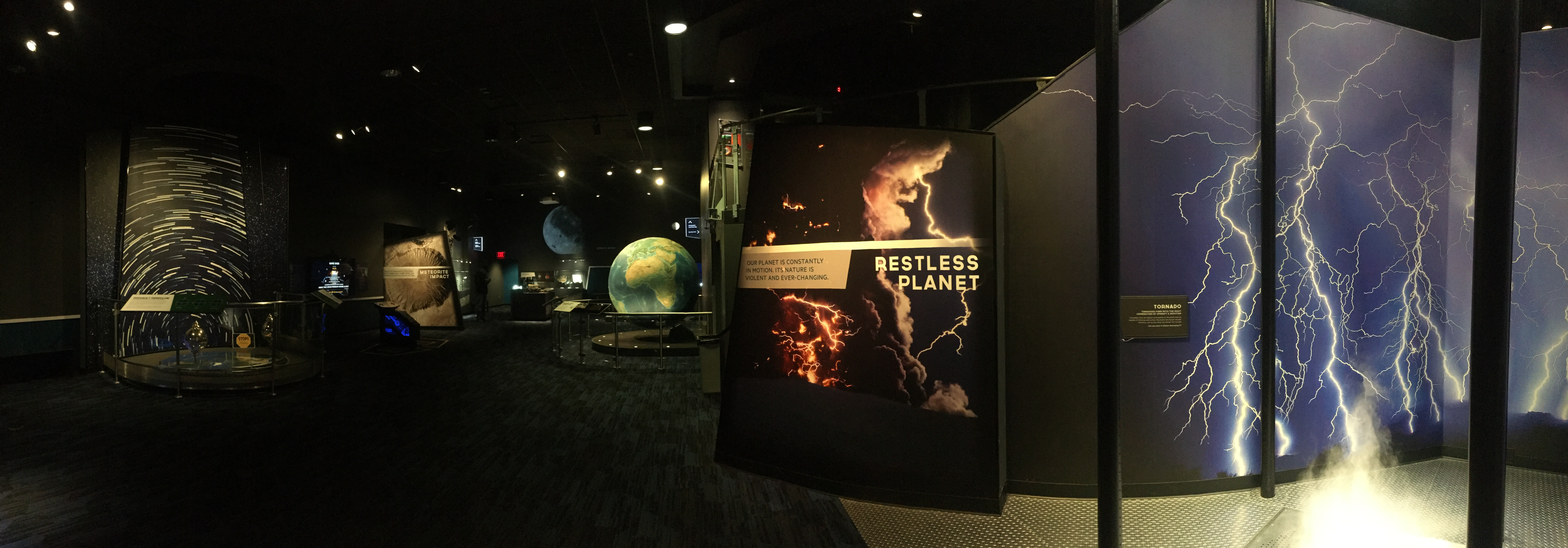The photograph captures a dimly lit section of a museum, predominantly featuring space and planetary exhibits. The ceiling is very dark, accentuated by several overhead lights. On the right-hand side, a prominent black sign with white text reads "Restless Planet," explaining that "Our planet is constantly in motion. Its nature is violent and ever-changing." The sign is illustrated with imagery of lightning and volcanic lava against its dark backdrop. To the left, a large globe prominently displays the continent of Africa. In the background, additional planet-themed displays are visible, including a meteorite exhibit and a portrayal of a black hole with arcing white lines. The most striking element on the right is a large image dominated by blue tones and streaking lightning. The overall setting is dim, with selective lighting emphasizing the various exhibits and creating a dramatic, educational atmosphere.